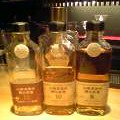The very small, approximately two-inch by two-inch image, appears to have been taken indoors in a dimly lit room, with a well-lit stage painted red in the background. Positioned on a small wooden table in the front and center are three clear glass bottles, all the same height, each with a black lid. The bottle on the right, full of a dark liquid, has a cream-colored label and a matching round label around its neck. The middle bottle, half-filled with a lighter liquid, has a similar black lid and white label. The third bottle on the left, nearly or completely empty, has a slightly darker brown label compared to the others. Additionally, the small size and blurriness of the photo make it difficult to discern the writing on the labels.